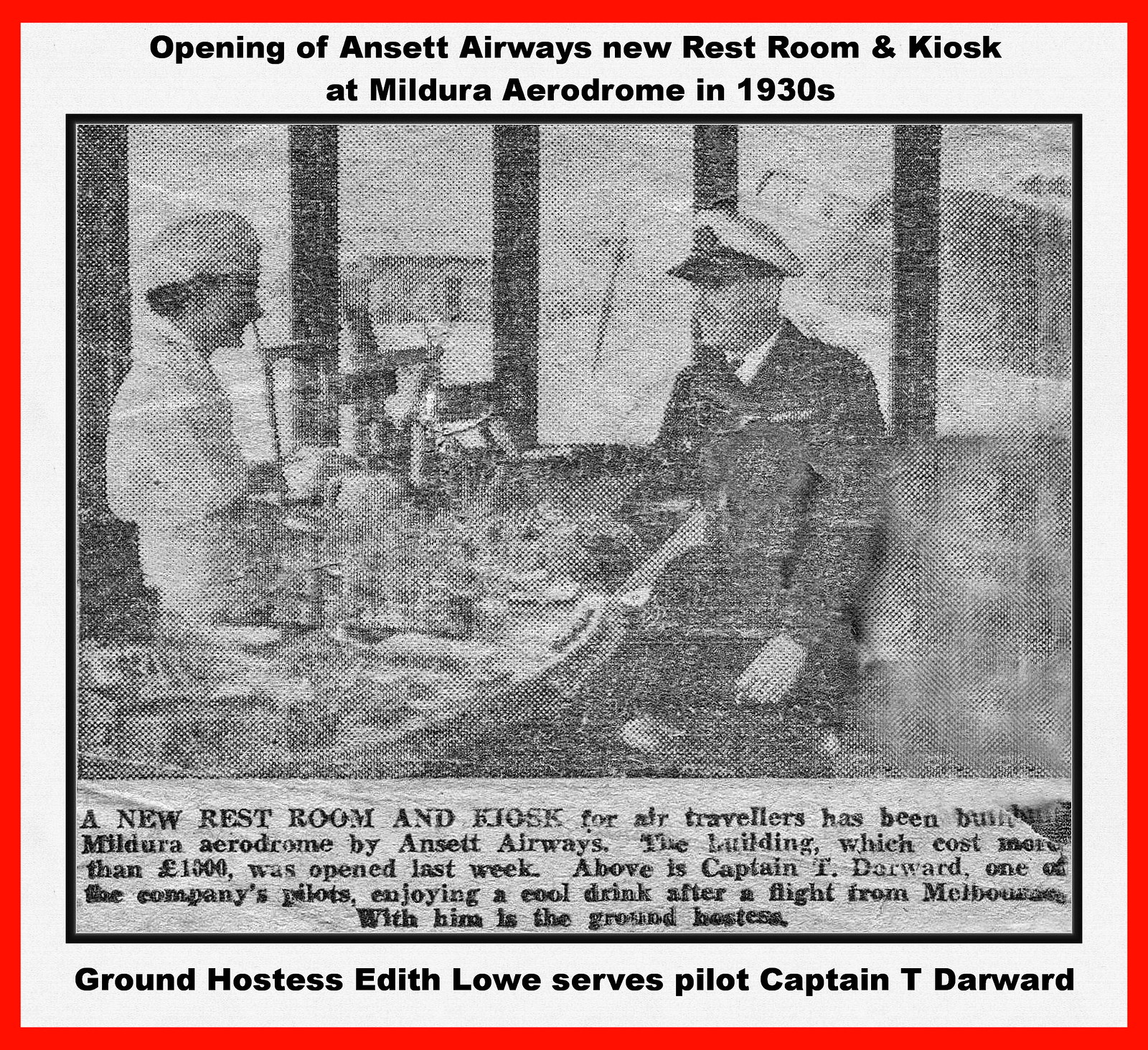A faded, black and white newspaper clipping from the 1930s, pasted onto a whiteboard and framed with a red box, features a vintage photograph commemorating the opening of Ansett Airways' new restroom and kiosk at Mildura Aerodrome. In the image, Captain T. Darward, a pilot dressed in a military uniform and hat, is seated at a small round table cluttered with items, enjoying a cool drink after a flight from Melbourne. To his left stands ground hostess Edith Lowe, donned in a white outfit and hat, serving him. The caption above the photograph mentions the opening of the new amenities, indicating the project's cost and its recent completion. Below the picture, the caption reads: "Ground hostess Edith Lowe serves pilot Captain T. Darward."